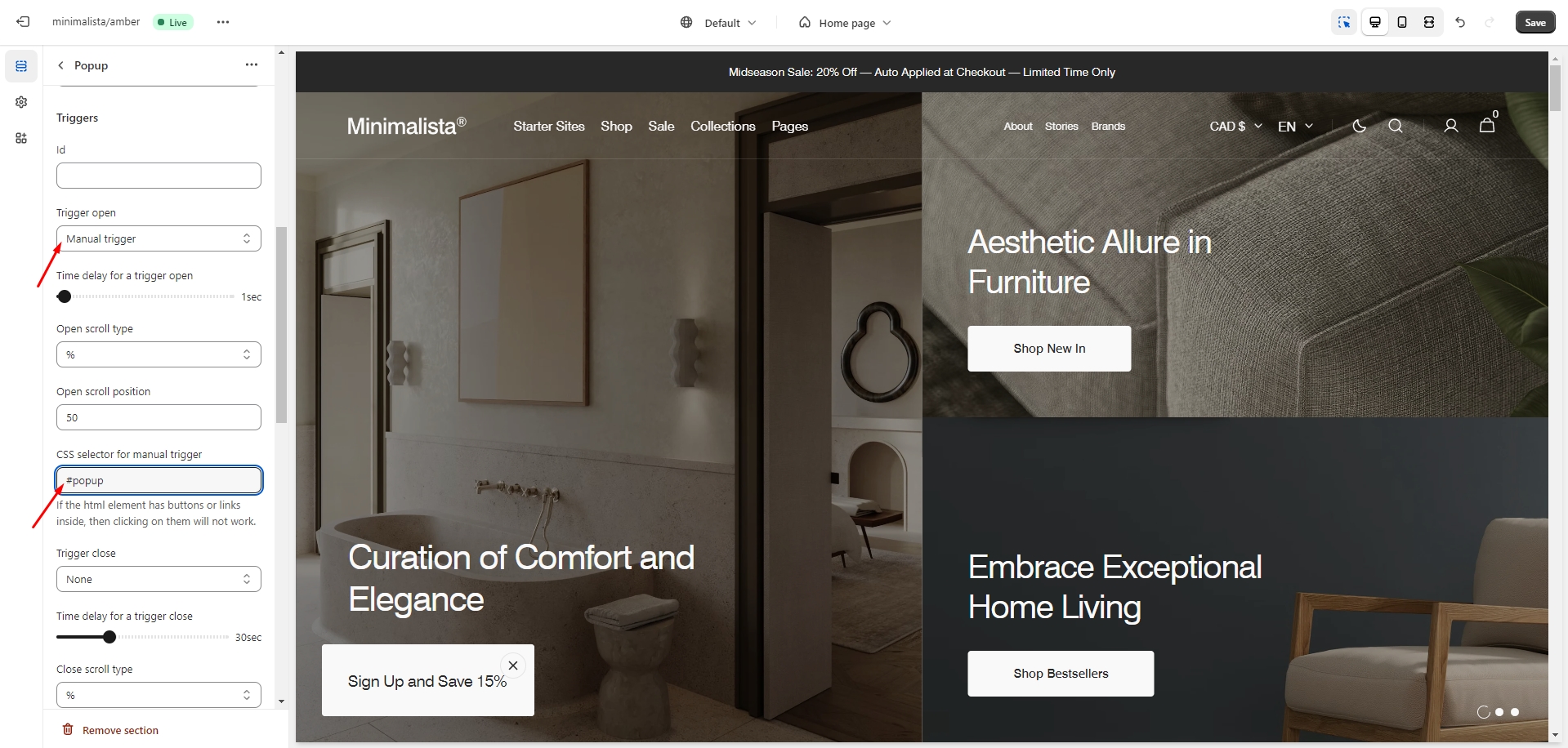This image captures a web page displayed on a computer screen. On the left-hand side, there is a prominent white section where a pop-up configuration interface is open. At the top of this interface, the label "Pop-up" appears, with sections labeled "Triggers" and "Trigger Open." A manually added red arrow points to the specific option "Manual Trigger." Below this, there are options labeled "Time Delay for Trigger Open" with a movable black dot along a dotted line, "Open Scroll Type," "Open Scroll Position," and a field for "CSS Selector for Manual Trigger," where a red arrow again highlights the text '#pop-up.'

The web page itself features the title "Minimalista" at the top, followed by navigational options such as "Starter Sites," "Shops," "Sale," "Collections," and "Pageo." At the bottom of the screen, the tagline "Curation of Comfort and Elegance" is prominently displayed. The main content showcases various interior design images, including a bathroom, a couch, and a chair. On the right side of the page, the text reads "Aesthetic Allure in Furniture," with the subheading "Embrace Exceptional Home Living" beneath it.